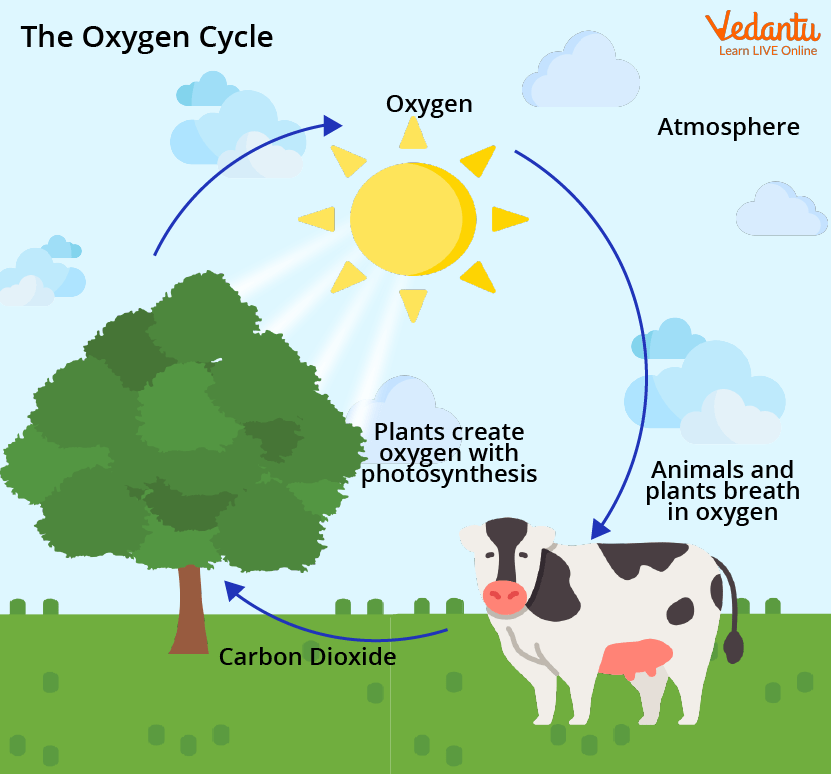The image depicts an illustrative, cartoony graphic designed to explain the oxygen cycle, likely aimed at children. At the top of the image, the title "The Oxygen Cycle" is written in black letters. The scene features a bushy green tree with a brown trunk on the left. To the tree's right stands a white cow with black spots, a pink nose, and pink udders, facing the viewer.

The cycle is depicted using blue arrows. One arrow starts from the cow and points left towards the tree, labeled "carbon dioxide." From the tree, another blue arrow rises to the yellow sun, which has triangular points and white rays, and is labeled "oxygen." A further blue arrow descends from the sun back towards the cow, with the text "animals and plants breathe in oxygen." The area beneath the sun, to the right of the tree, contains the text "plants create oxygen with photosynthesis." The top right corner of the image includes the word "atmosphere." Beyond these details, the uppermost right corner features the phrase "Divine Online" in orange cursive letters. The entire illustration is placed over a green grassy ground, enhancing its family-friendly, educational design.